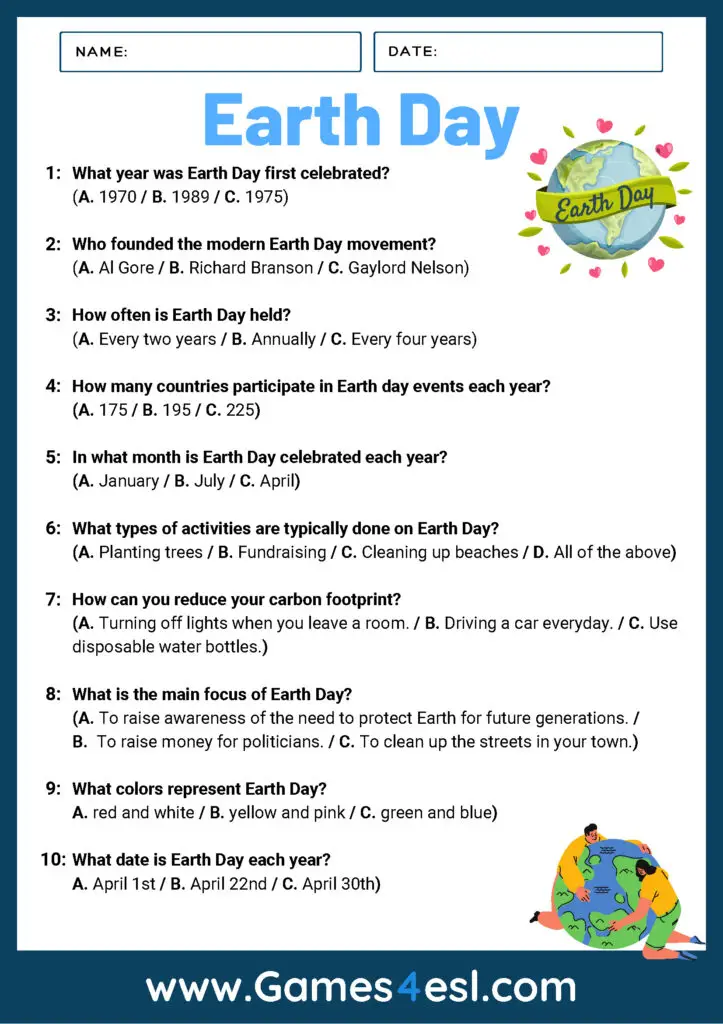This poster is dedicated to Earth Day and features a quiz to educate viewers on various facts about the event. At the top, it prominently displays the title "Earth Day" followed by a series of questions related to the environmental celebration. 

1. **What year was Earth Day first celebrated?**
   - A. 1970
   - B. 1989
   - C. 1975

2. **Who founded the modern Earth Day movement?**
   - A. Al Gore
   - B. Richard Branson
   - C. Gaylord Nelson

3. **How often is Earth Day held?**
   - A. Every two years
   - B. Annually
   - C. Every four years

4. **How many countries participate in Earth Day events each year?**
   - A. 175
   - B. 195
   - C. 225

5. **In what month is Earth Day celebrated each year?**
   - A. January
   - B. July
   - C. April

6. **What types of activities are typically done on Earth Day?**
   - A. Planting trees
   - B. Fundraising
   - C. Cleaning up beaches
   - D. All of the above

7. **How can you reduce your carbon footprint?**
   - A. Turning off lights when you leave a room
   - B. Driving a car every day
   - C. Using disposable water bottles

8. **What is the main focus of Earth Day?**
   - A. To raise awareness of the need to protect the Earth for future generations
   - B. To raise money for politicians
   - C. To clean up your streets and town

9. **What color represents Earth Day?**
   - A. Red and white
   - B. Yellow and pink
   - C. Green and blue

10. **What date is Earth Day each year?**
    - A. April 1st
    - B. April 22nd
    - C. April 30th